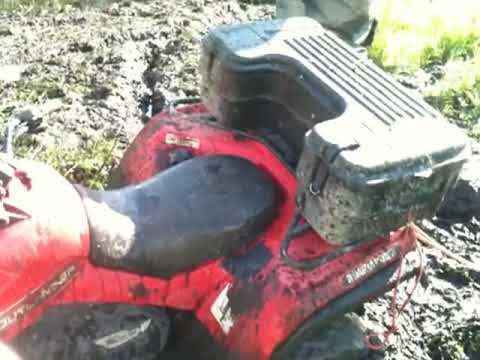The image is a color photograph of a red off-road vehicle, likely either an ATV or a three-wheeler, taken outside during the day under bright sunlight. The vehicle, which has a black seat and black detailing, is positioned with its rear end in the center of the frame and pointed to the left, with the steering also angled to the left. The front wheel is not visible as it's cut off by the edge of the photograph. Behind the seat is a black plastic case or toolbox, equipped with straps, ideal for carrying tools or other items. The terrain around the vehicle is predominantly muddy, suggesting it has been driven through thick, wet mud, as evidenced by the mud splattered on the ATV itself. A small patch of grass can be seen in the upper right corner of the image, lit up by the bright sunlight. The background also includes an obscure object, although the primary focus remains on the muddy, red off-road vehicle.